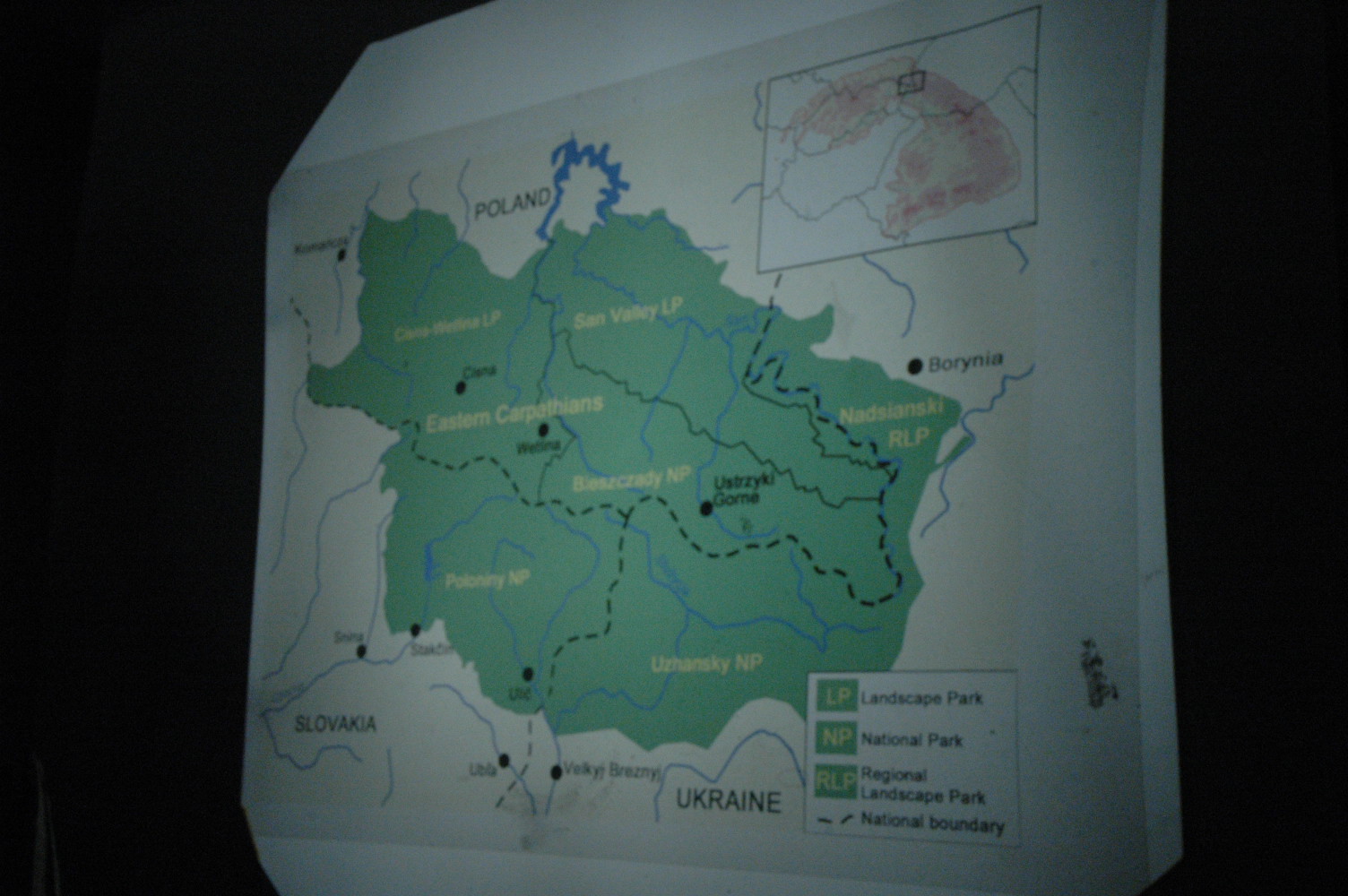The image depicts a map shown on a black background, likely projected on a screen, highlighting an area at the intersection of Poland, Slovakia, and Ukraine. The map features various green-shaded regions and intricate, jagged lines in blue and green, indicating different types of parks and boundaries. Labels in different shades of green identify specific areas, although the small, light green text is difficult to read. The upper right and lower right corners contain a key with green squares and yellow font, explaining the acronyms: LP for Landscape Park, NP for National Park, and RLP for Regional Landscape Park. The map also marks National Boundaries with jagged lines.